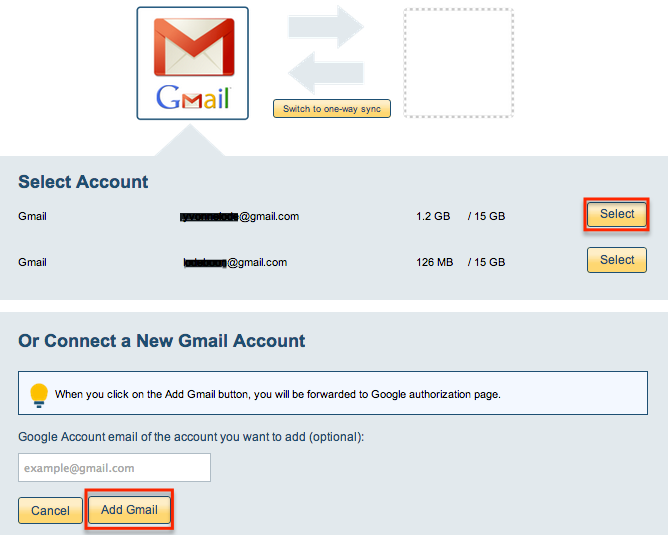The image showcases a webpage interface related to Gmail account sync settings. In the top left corner, there is a sizable square icon featuring the Gmail logo. The logo includes the classic Gmail colors: the "G" in purple, "M" in red, "a" in yellow, "i" in blue, and "l" in a blue-green shade.

Directly to the right of the logo are two arrows stacked vertically: the top arrow points to the right, while the bottom arrow points to the left. Below the left-pointing arrow, there is a yellow block with the text "Switch to one-way sync."

To the immediate right of this block and arrows, an empty gray square is displayed. Beneath this setup, the text "Select account" appears, followed by a redacted Gmail address ending in "@gmail.com."

To the right of the redacted email address is the "Select" button. Further down, the interface prompts users to either connect an existing Gmail account or add a new one. The options "Add Gmail" and "Cancel" are located at the bottom of the interface.